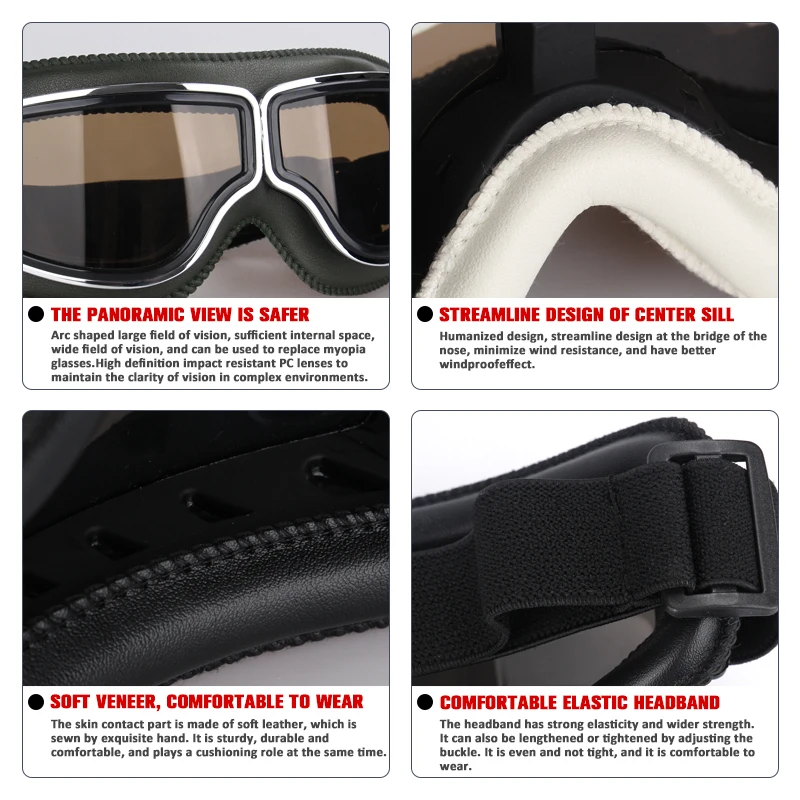The image is a detailed breakdown of goggles, presented in a grid of four sections on a plain white background, each bordered with a thin black pinstripe outline. Each section contains a close-up of different parts of the goggles and descriptive text beneath.

In the top left section, we see the front of the goggles. The accompanying text reads, "The panoramic view is safer" in red, followed by detailed features in black: "Arc-shaped, large field of vision, sufficient internal space, wide field of vision, and can be used to replace myopia glasses. High-definition impact-resistant PC lenses maintain clarity of vision in complex environments."

The top right section highlights a close-up of the bridge of the nose area of the goggles. The red text states, "Streamlined design of center sill," with the black text explaining, "Humanized design, streamlined at the bridge of the nose, minimizes wind resistance, and has a better windproof effect."

In the bottom left section, there is an up-close image of the soft black portion that contacts the skin. The red text here reads, "Soft veneer, comfortable to wear," and the black text adds, "The skin contact part is made of soft leather, sewn by exquisite hand, making it sturdy, durable, and comfortable while providing a cushioning effect."

The bottom right section shows a close-up of the headband. The red text says, "Comfortable elastic headband," and the detailed black text elaborates, "The headband has strong elasticity and wider strength. It can be lengthened or tightened by adjusting the buckle. It is even and not tight, ensuring comfort during wear."

Overall, the image meticulously explains each functional aspect of the goggles, emphasizing safety, comfort, and performance-enhancing features.